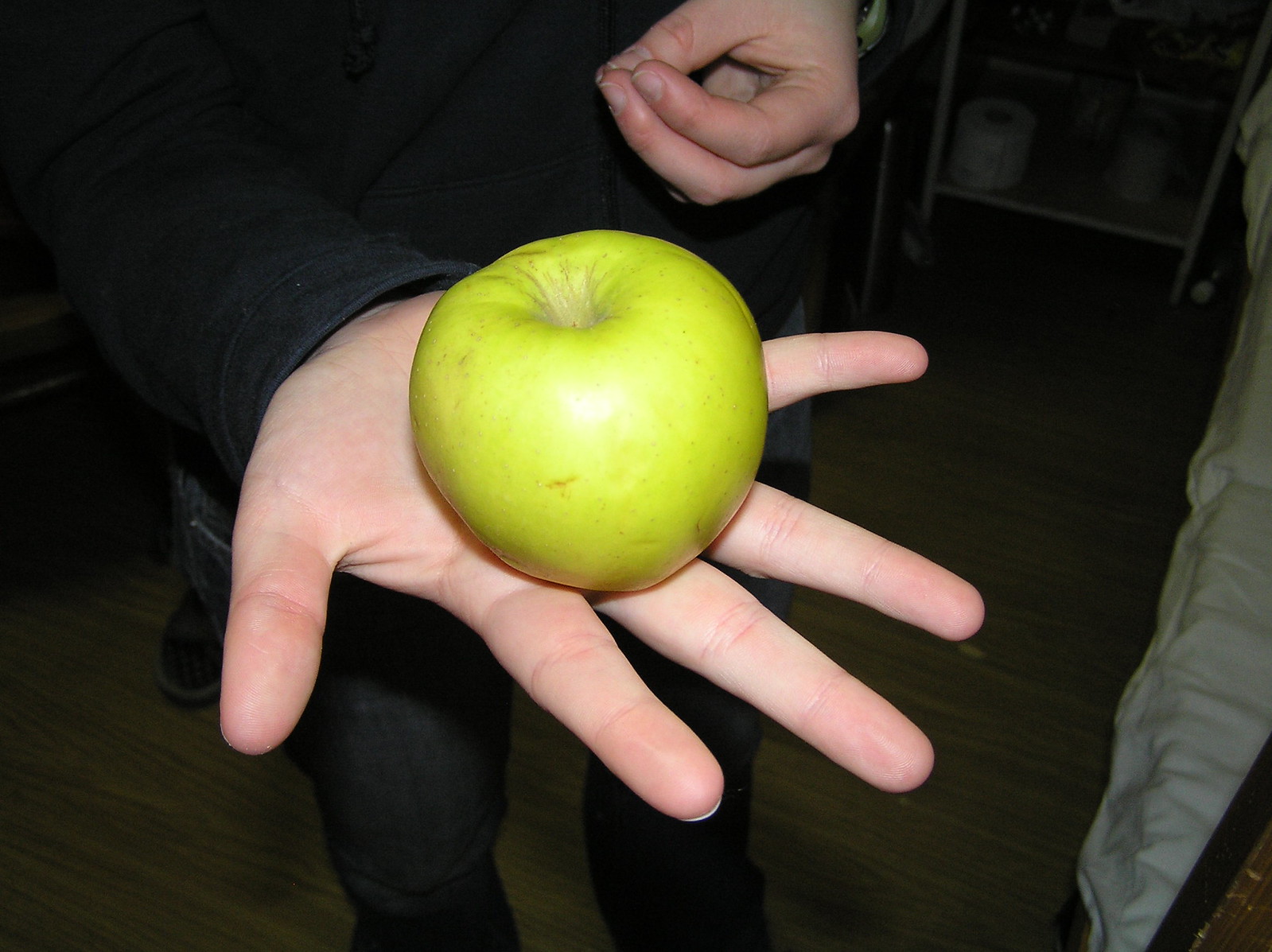In this close-up photograph with dim lighting, the central focus is on a white, male hand held palm up, fingers splayed, presenting a green apple resting in the middle of the palm. The apple has a few minor imperfections dotting its surface. The man's arm, clad in a long-sleeved black denim jacket, extends forward. He is dressed in very dark blue jeans, and his other hand is held close to his body, with the thumb resting on the tips of his first two fingers. In the background to his right, a wooden footboard of a bed with white sheets is visible, against a floor of dark stained wood. Additionally, behind the man, part of another person's leg wearing a dark chocolate brown lace-up boot can be seen, adding a subtle layer of depth to the scene.